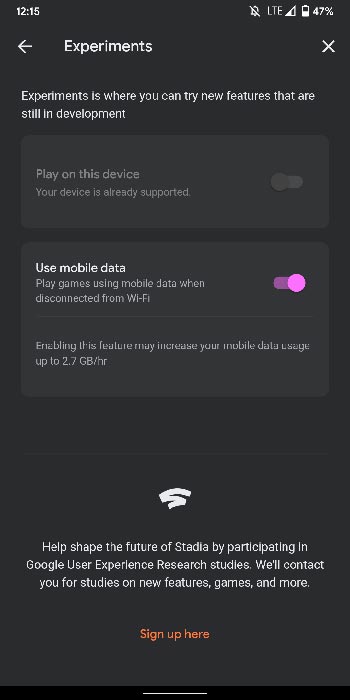The image depicts an Android device screen displaying the "Experiments" section of an app. In this section, users can try out new features currently in development. One of the features highlighted is "Play on this device," which is grayed out, indicating it is not available for use. Another feature, "Use mobile data," is enabled, with a purple switch signifying its active status; this allows users to play games using mobile data when disconnected from Wi-Fi, though enabling this feature may increase data usage up to 2.7 gigabytes per hour.

At the bottom of the interface is the Stadia logo. A message encourages users to help shape the future of Stadia by participating in Google user experience research studies. Interested users are invited to sign up via a red "Sign up here" link. The overall interface features a dark gray background with white text, creating a clean, modern aesthetic.